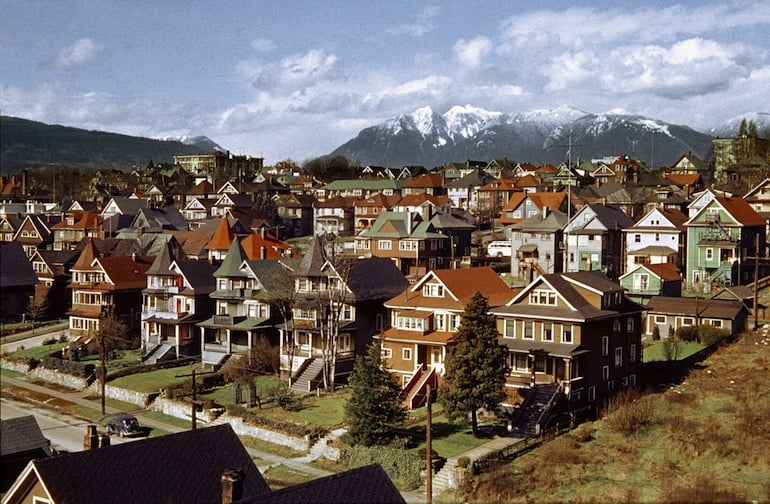This horizontal rectangular photograph captures a picturesque landscape, dominated by a serene blue sky adorned with fluffy white clouds in the top third of the image. The right side of the background showcases majestic, snow-capped mountains that provide a stunning contrast to the vibrant scene unfolding below.

In the bottom two-thirds of the photograph, a quaint, charming town unfolds, characterized by rows of Victorian-style houses. These houses, mostly three stories tall, line the streets in neat rows, creating a harmonious pattern of architecture. The houses are painted in a palette of muted yet inviting colors—green, brown, and gray—each complemented by well-manicured green lawns.

To the left, a factory building peeks through, offering a subtle hint of the town's industrial roots. However, the primary focus remains on the residential streets stretching out in a picturesque tableau, complete with front porches and steps leading up to welcoming doorways. Some of the houses feature distinctive cone-shaped rooflines, adding a unique flair to the overall architectural charm.

In the bottom right corner of the photograph, a patch of brushy area with green and brown vegetation adds a touch of wild, natural beauty to the otherwise well-kept scene. The streets are clean and orderly, reflecting the care and pride of the town's residents. This image captures the essence of a beautifully maintained town nestled comfortably at the base of awe-inspiring mountains, offering a perfect blend of natural wonder and architectural elegance.